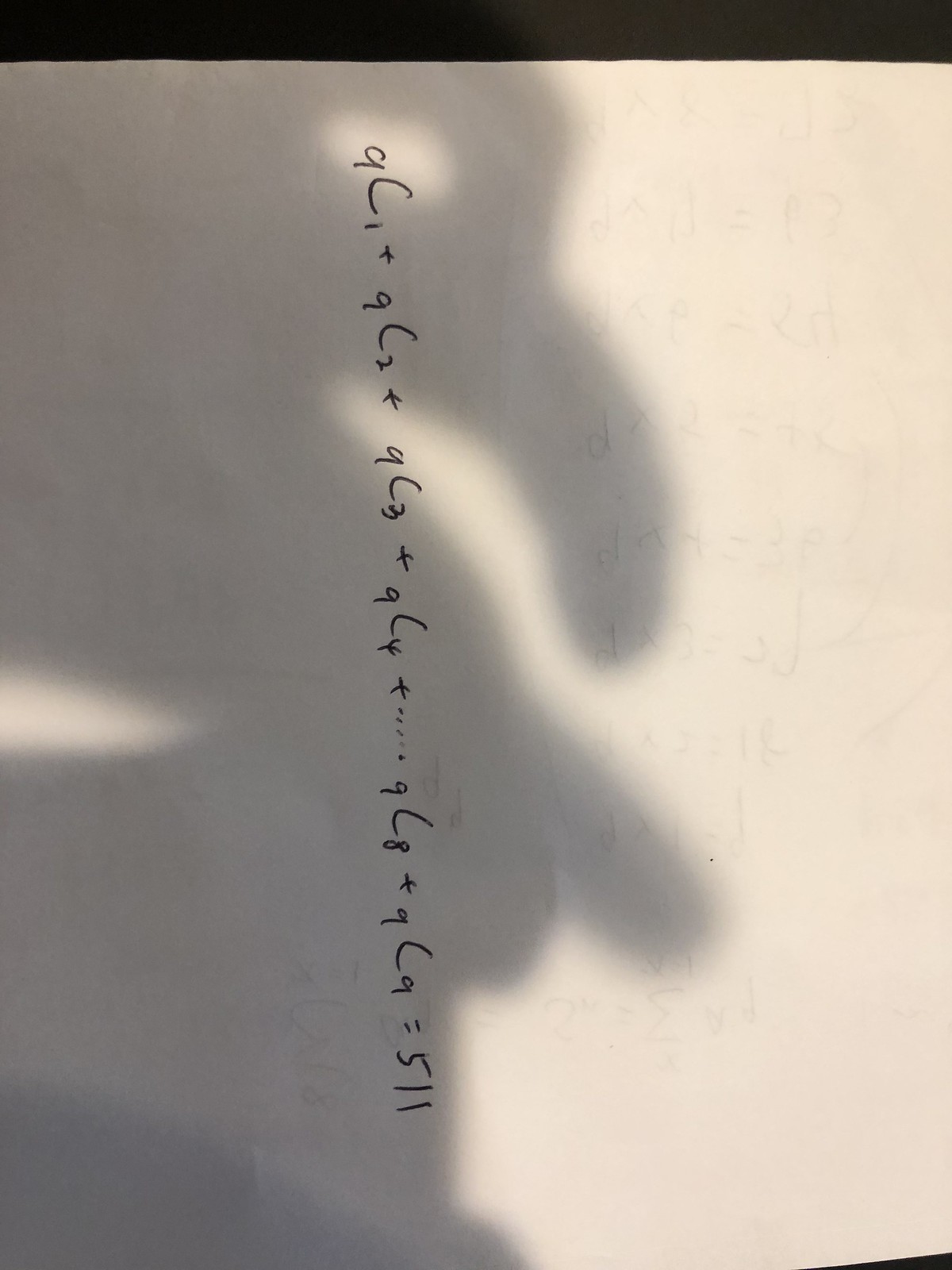This photograph captures an extensive math problem written on the back side of a piece of paper, with numbers and equations faintly visible from the opposite side, indicating a densely filled sheet. The math problem is composed of a series of vertical numbers and symbols located in the center of the paper, written either in black ink or a regular No. 2 pencil. The sheet is oriented horizontally, requiring the viewer to tilt their head to the right to read the problem correctly. The vertical sequence begins with the numeral nine and proceeds with a combination of letters, commas, and plus signs, resembling the notation for combinations in mathematics. The sequence starts with "9C," followed by "9C2," "9C3," continuing in this manner until "9C9," and concluding that the series equals 511. Additionally, the shadow of the person taking the picture is visible, including their left hand holding the camera, adding a candid, behind-the-scenes feel to the image.